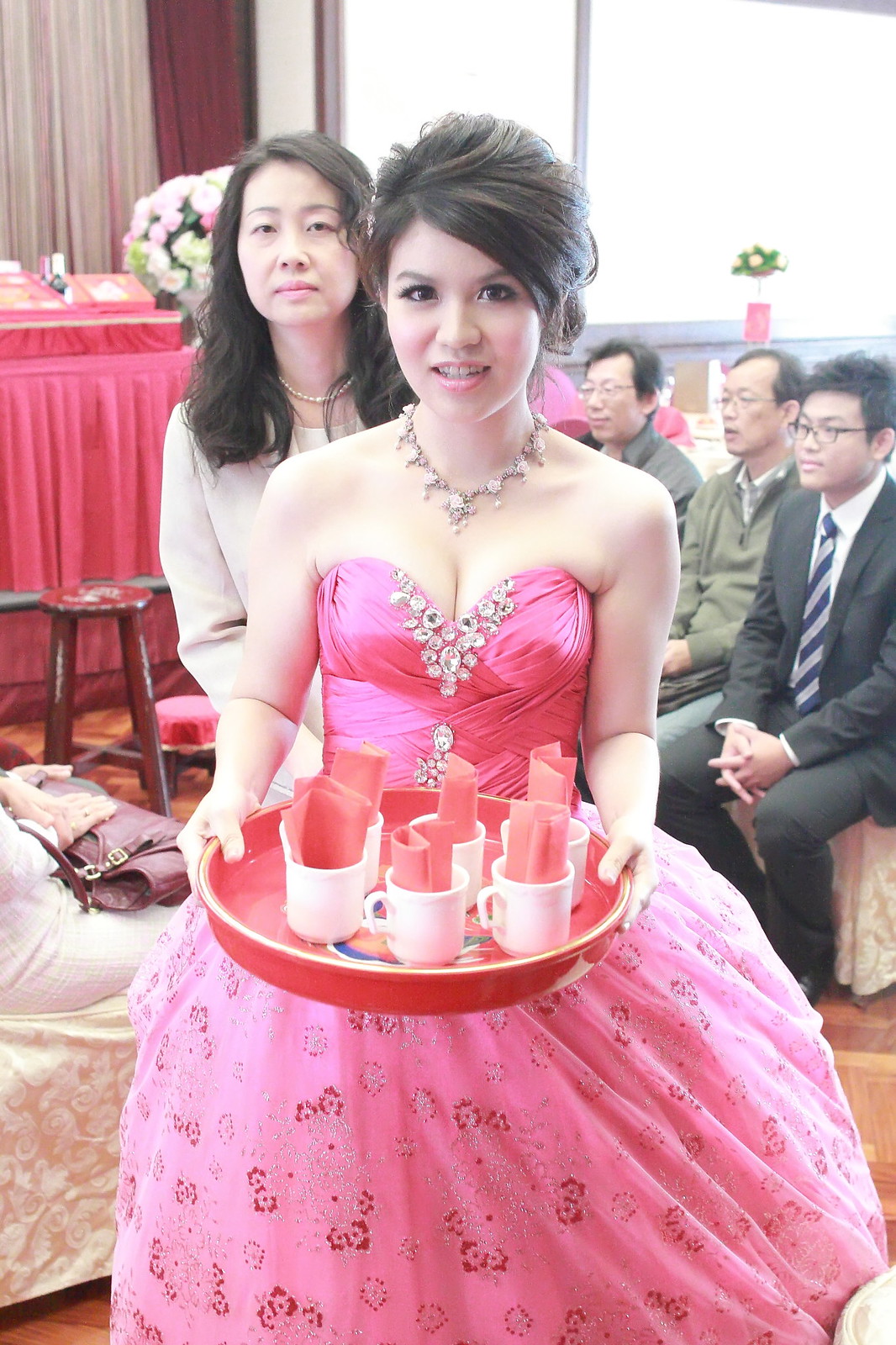In this brightly lit indoor photo taken during the daytime, a young woman in a striking pink, poofy, sleeveless dress adorned with white faux diamond jewels is the central focus. The dress features intricate designs of red and white flowers at the bottom, making it resemble a princess gown. The young woman, who has brown hair and wears a silver necklace, is holding a red circular tray with six white teacups, each containing a pink napkin. She gazes directly into the camera with a calm expression.

Behind her to the left stands an older woman, possibly her mother, with similar brown hair, wearing a white suit, a pearl necklace, and a tan overcoat. This woman also looks straight into the camera. In the background to the right, three men sit beside a woman with a red purse on her lap. The men appear older, with some having receding hairlines, and all wear glasses. One man is in a black suit with a white shirt and a blue and white striped tie, another in a greenish sweater, and the third in a grey vest-like outfit.

The setting includes a large window with bright light streaming through it, obscuring any clear view outside. Next to the window is a vase with a green plant, and the window is framed by reddish and pinkish-white curtains. Additionally, there are white silk paisley-design sofas visible in the background, a bouquet of flowers, a podium draped in pink fabric, and a lady with her hands on a purse. The overall atmosphere suggests a festive and elegant gathering.